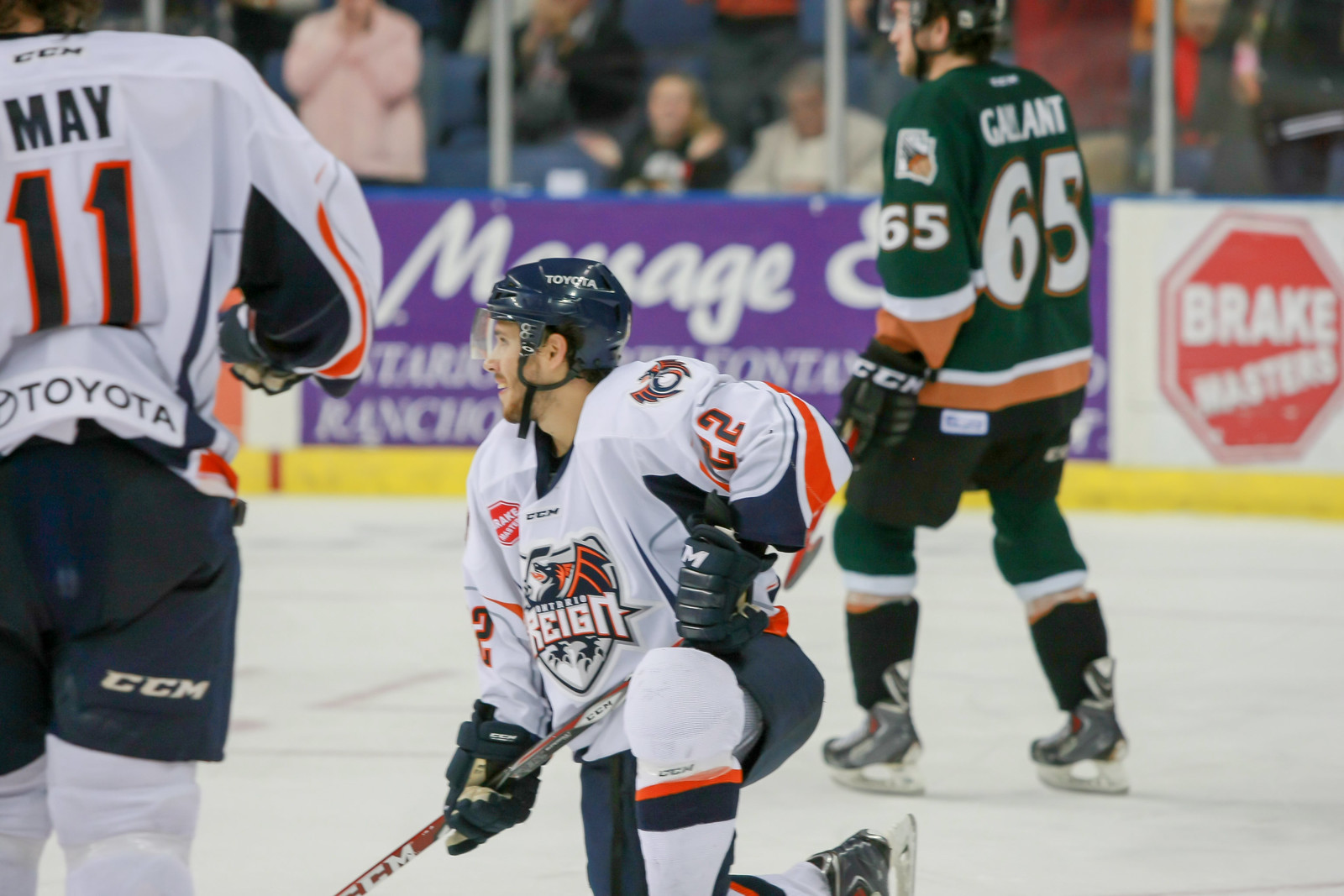The photo captures an intense moment during a professional or college hockey game, featuring three players on the ice. Two players are in white uniforms, labeled with "Rain" and a griffin mascot. One of these players, with the number 11 and the last name "May" on his jersey, has "Toyota" listed as a sponsor on the back. The third player, dressed in a green jersey with the number 65, represents the opposing team, "Gallant." The player in the foreground, wearing number 22, is kneeling down and holding a hockey stick, showcasing the "Rain" team’s dragon logo on his jersey. The scene is set against a background of out-of-focus spectators and various advertisements along the rink's fence, including a prominent purple banner for Massage Envy and another for Break Masters. The players' dynamic positions and the vivid details of their uniforms and gear immerse the viewer in the live action of the game.